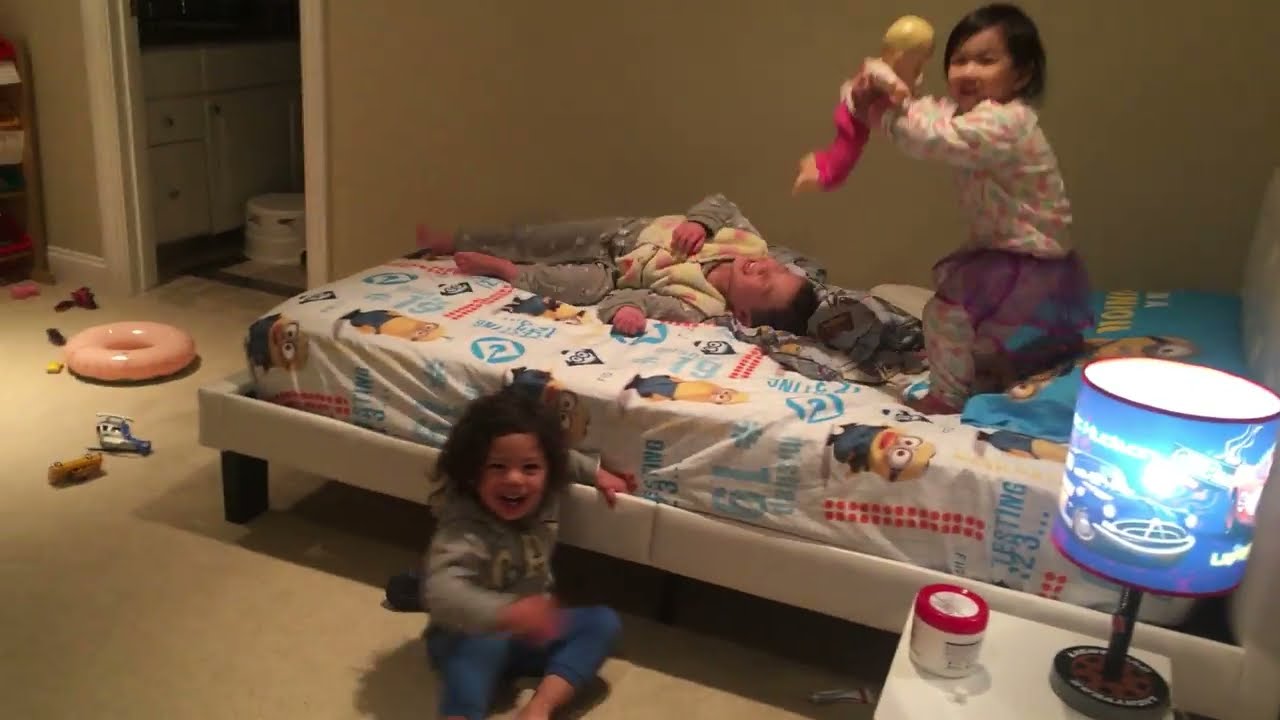In a lively, well-lit kid's bedroom, three toddlers are immersed in play. The central focus is a bed adorned with cartoon Minion bed sheets and a matching blue pillow. One toddler, wearing a pink and green shirt with gray pants, stands exuberantly on the bed, clutching a blonde doll in red pants. To her left, another toddler, dressed in a gray shirt with gray pants, is lying down on the bed, laughing joyously with one hand on his chest and the other flung to the side. On the floor to the left of the bed sits the third child, with black hair and a gray shirt paired with black pants, smiling directly at the camera. Nearby, the bedroom features a side table with a black lamp topped with a blue lampshade and a white container with a red lid. Scattered toys lie on the brown carpet, and an inflatable donut rests at the foot of the bed. The background reveals a beige wall and an open entryway leading to an adjacent room. The scene captures a moment of pure childhood delight and energy.